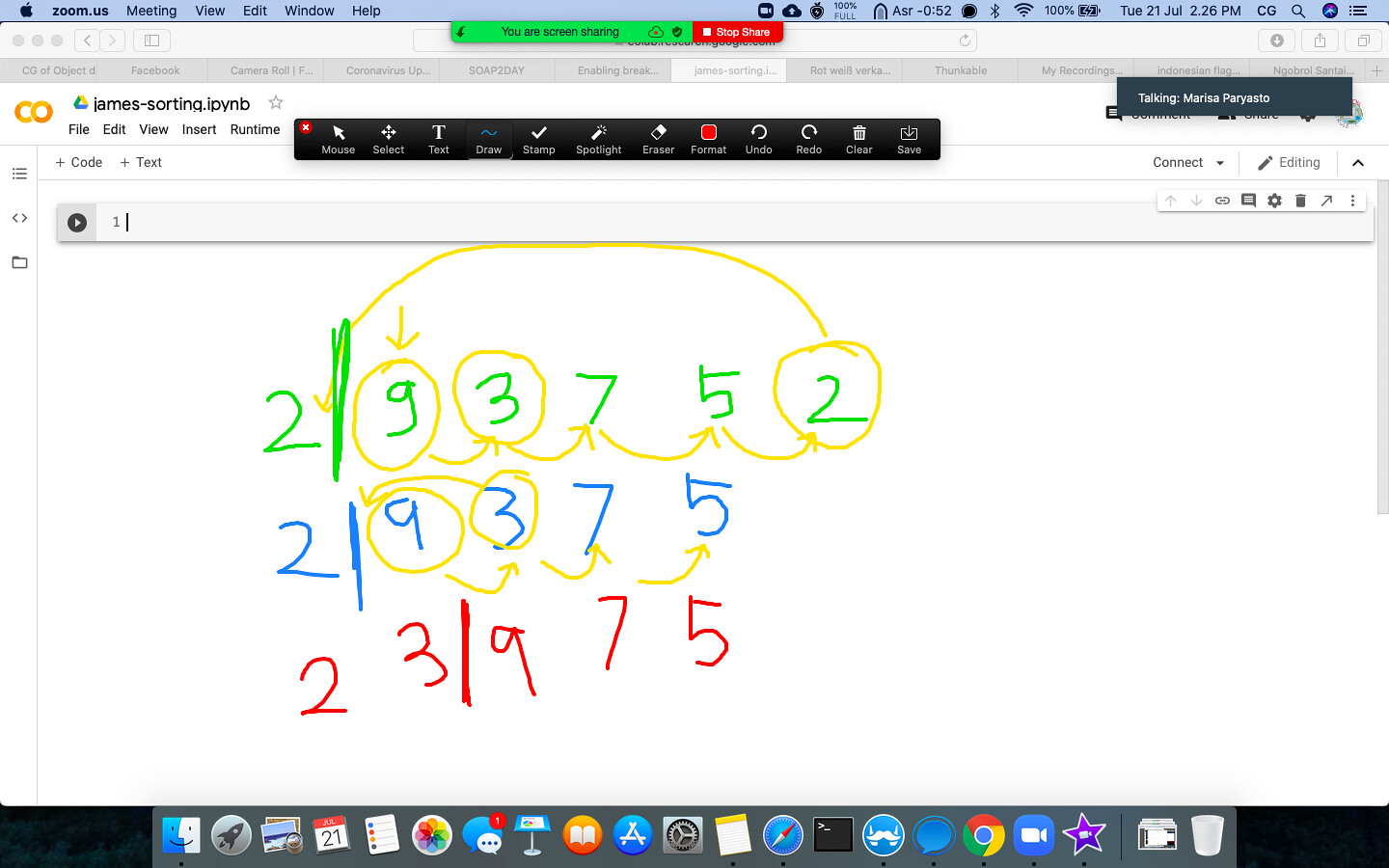A detailed description of the image would be as follows:

This image depicts a child's math homework being worked on via a Zoom.us session. The digital workspace, presumably belonging to a student named James, showcases a specific sorting or problem-solving activity related to mathematical sequences or operations. The activity appears to be divided into three distinct lines, each with different colored annotations and marked with the date and time.

1. **First Line (Green)**: The sequence starts with "2 / 9" (where the character "9" could potentially be a "G"), followed by "3", "7", "5" with continuous arrows connecting each number. The numbers "2", "9"/"G", and "3" are circled in yellow.

2. **Second Line (Blue)**: This sequence is formatted as "2 / 9 3 7 5". Arrows under each number link them together, resembling a pathway. Here, the numbers "9" and "3" are highlighted in yellow circles.

3. **Third Line (Red)**: The final line reads "2 3 / 9 7 5". This line contains no circled numbers and is solely annotated in red.

The entire activity is marked by a series of arrows and circles in yellow to emphasize connections and important points in the sequence. The use of color coding (green, blue, and red) for the lines likely indicates different stages or parts of the problem. This meticulous layout suggests that James is either solving a complex problem or organizing numbers in a meaningful way to understand a mathematical concept better.